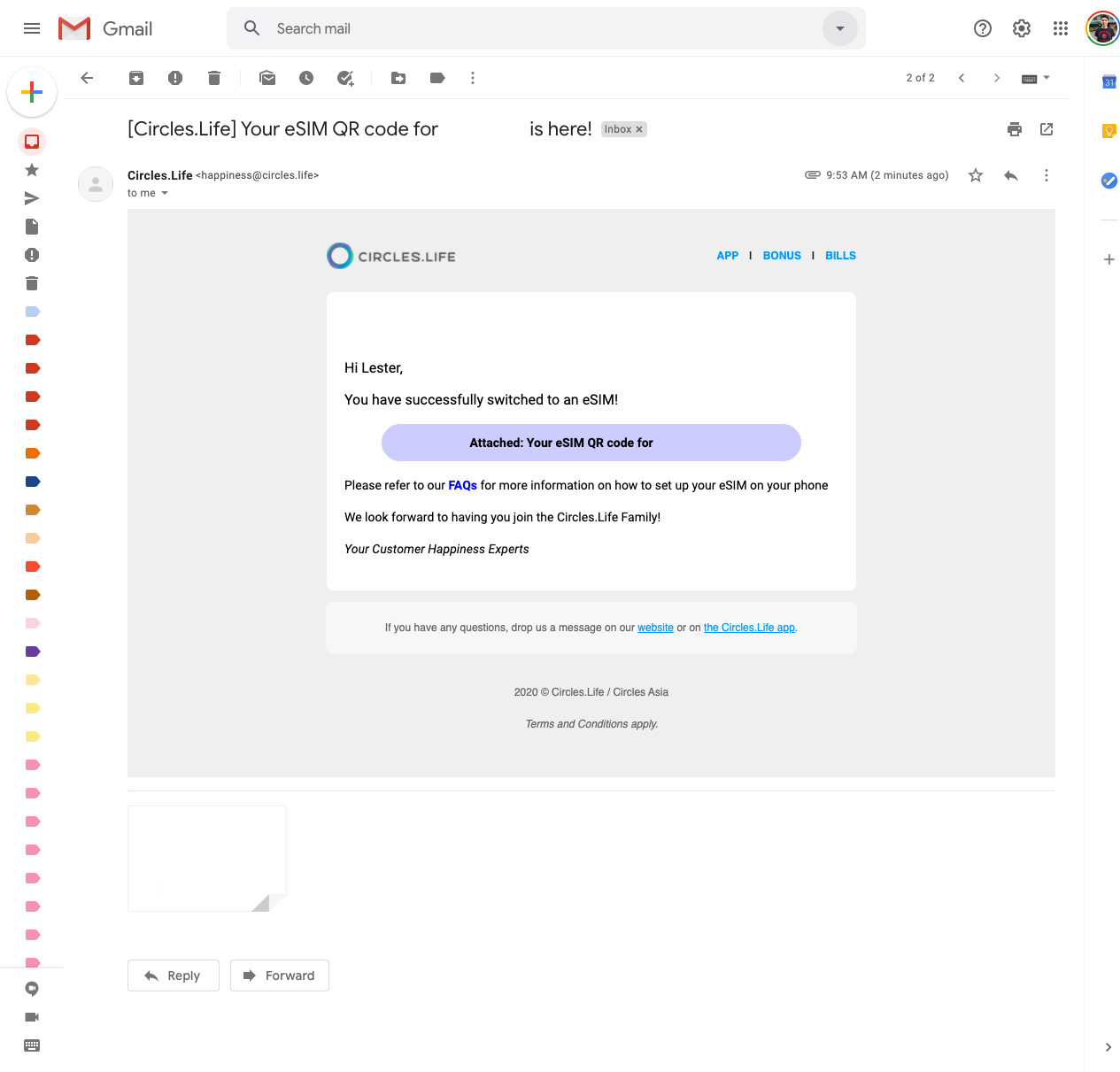The screenshot displays a webpage, specifically an email from Gmail. At the top of the page, the Gmail logo is visible alongside a search bar, a question mark icon, a settings gear icon, a grid icon representing Google Apps, and the recipient's profile picture. 

The email is titled "Circles.life: Your eSIM QR Code for [Blank] is Here." The sender's address, "Circles.life," appears twice at the beginning, accompanied by a logo consisting of a circle with various shades of blue.

On the right side of the email, there are links labeled "App," "Bonus," and "Bills." The body of the email begins with a greeting: "Hi Lester, you have successfully switched to an eSIM." Below the greeting is a prominent purple oblong button. The text on the button instructs: "Attached is your eSIM QR code for [Blank]. Please refer to our FAQs for more information on how to set up your eSIM on your phone. We look forward to having you join the Circles.life family. Your Customer Happiness Experts."

At the bottom of the email, a message reads: "If you have any questions, drop us a message on our website or on the Circles.life app." Along the side of the page, various flags and stars in different colors are visible, indicating the different labels and categories available for organizing emails.